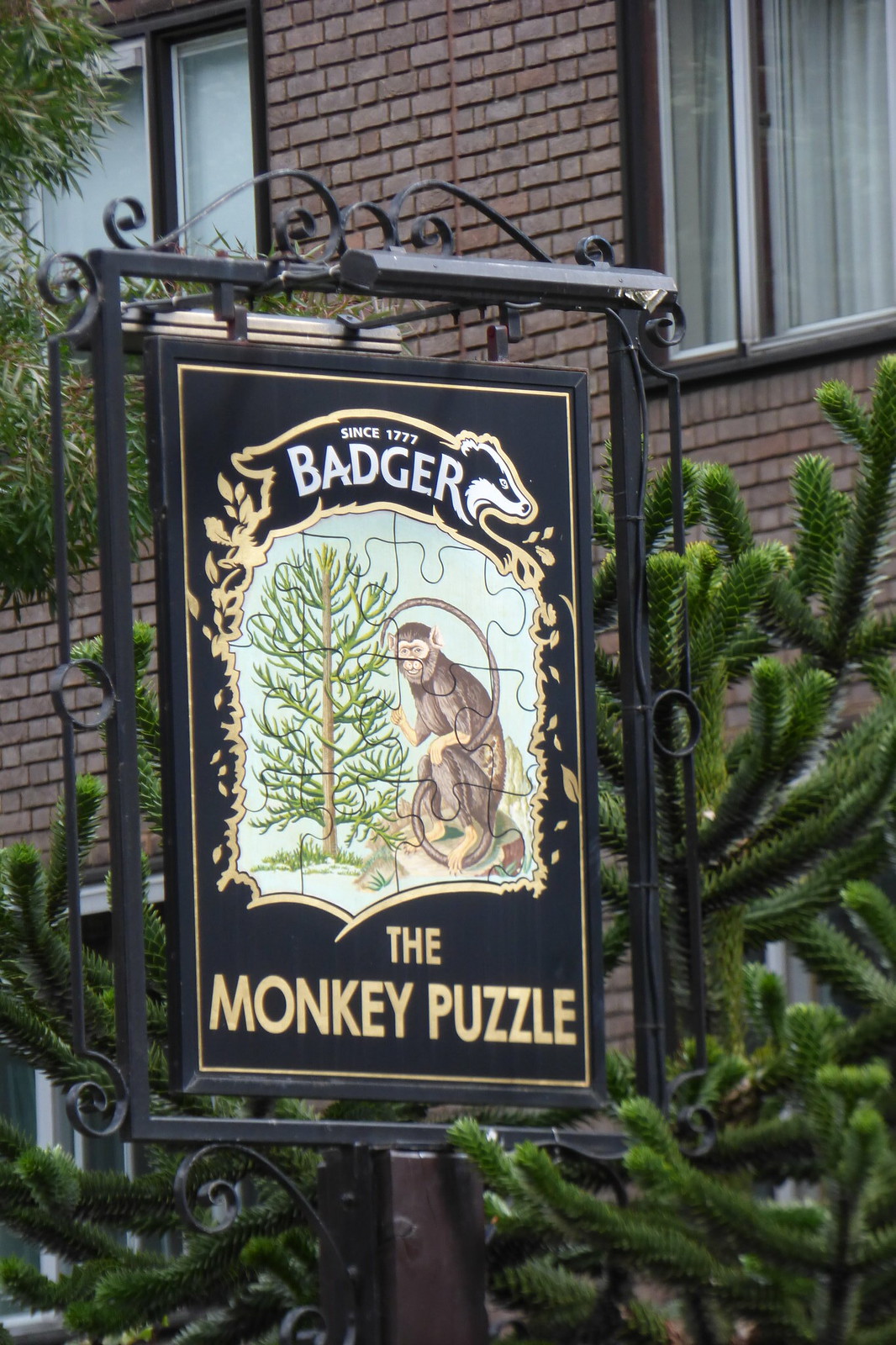In the outdoor photograph, there's a beige brick apartment building in the background with two uniformly spaced windows. The right window has light-colored, striped drapes, while the left window features a rolled-up blind. In front of the building, several evergreen shrubs are visible. The central focus of the image is an ornate, black scrolled cast iron sign mounted into the ground. The sign, with gold feathering, has an outline of a badger at the top with the text "Since 1777, Badger." Below the badger illustration, it reads "The Monkey Puzzle," flanked by an image resembling a jigsaw puzzle, depicting a monkey next to a Monkey Puzzle tree. This tree mirrors the smaller Monkey Puzzle tree located to the right of the sign, which is characterized by its slim, green branches. Another green tree is partially visible towards the top left of the photograph, adding more greenery to the scene. The detailed, pub-like sign creates a charming focal point against the backdrop of the structured apartment building and surrounding vegetation.